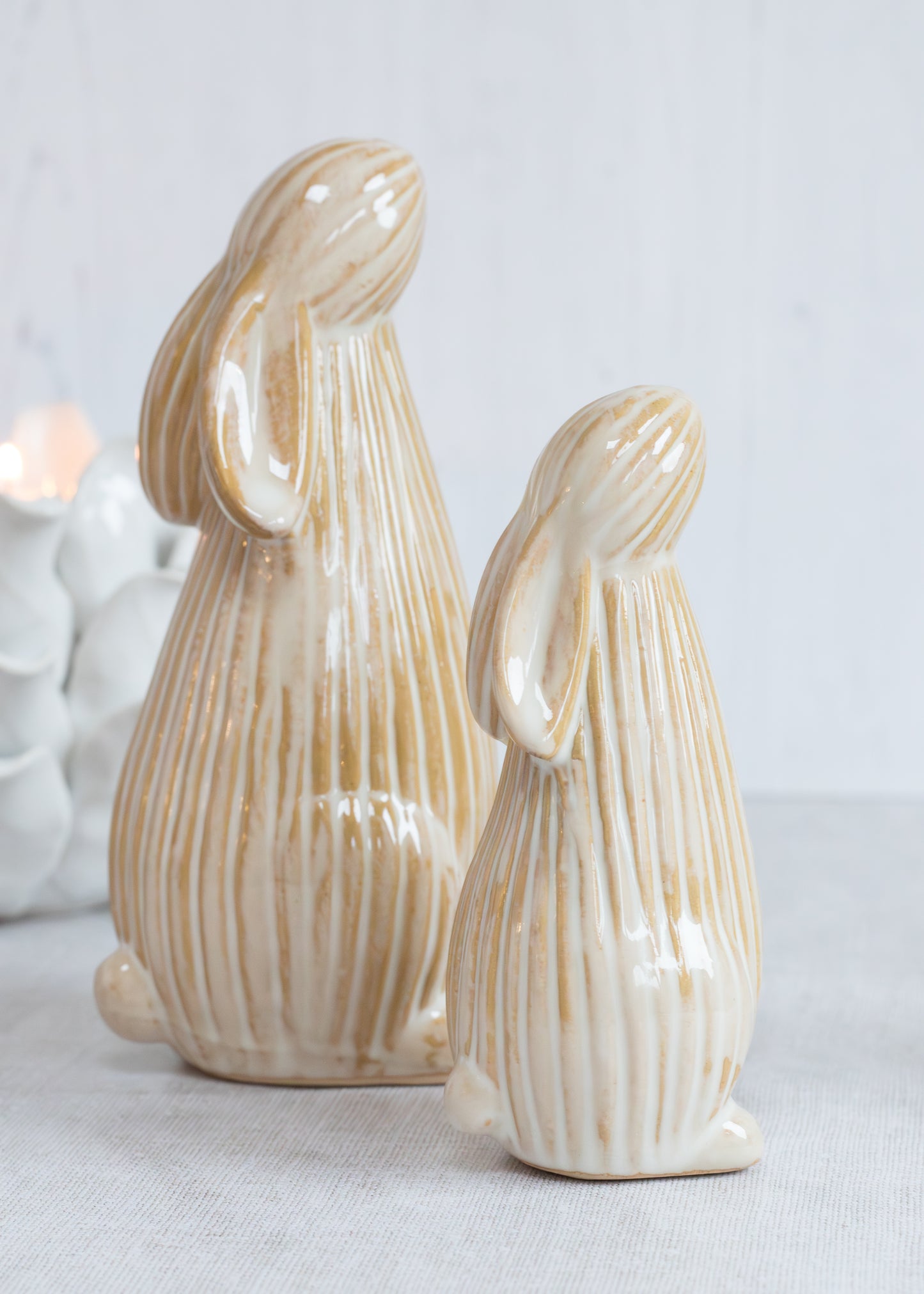This photo features a pair of adorable ceramic bunny sculptures positioned against a soft neutral white backdrop. Both bunnies, one slightly larger than the other, are sculpted with long, slender bodies and elongated necks that culminate in small heads looking upward, their long ears draping elegantly behind them. The surface they rest on appears to be a white cloth or carpet. Each bunny boasts reflective surfaces with subtle beige stripes down the center, capturing and highlighting glimmers of light. The bunnies lack detailed appendages, presenting a smooth, cartoon-like aesthetic, reminiscent of salt shakers in their size and simplicity. In the background, there are hints of white objects, possibly teacups, adding to the overall serene and neutral ambiance of the scene.